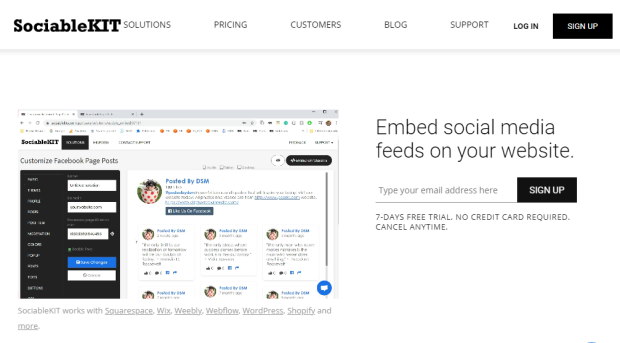This screenshot, taken from the SociableKit website, showcases their service designed for embedding social media feeds onto a website. Positioned at the top left is the SociableKit logo, while the top right corner features navigation links labeled "Solutions," "Pricing," "Customers," "Blog," "Support," "Login," and a prominently highlighted "Sign Up" button in black.

Dominating the left section of the main content area is a screenshot of the SociableKit interface. This interface demonstrates the customization options available for embedding a Facebook page post feed, allowing users to adjust the appearance and settings of their Facebook feed. The depicted Facebook feed includes multiple posts featuring profiles, pictures, names, and content.

A large headline above the screenshot reads, "Embed Social Media Feeds on Your Website." Directly below this headline, a text box invites users to "Type your email address here" accompanied by a black "Sign Up" button. Further down, an additional text box notes, "Seven days free trial, no credit card required."

At the bottom, there's information emphasizing that SociableKit is compatible with various website builders and platforms such as Squarespace, Wix, Weebly, Webflow, WordPress, Shopify, and more. The overall design is clean and modern, characterized by a white background and black accents, making the website user-friendly and visually appealing. The inclusion of a screenshot serves to effectively demonstrate the functionality and layout of the service.